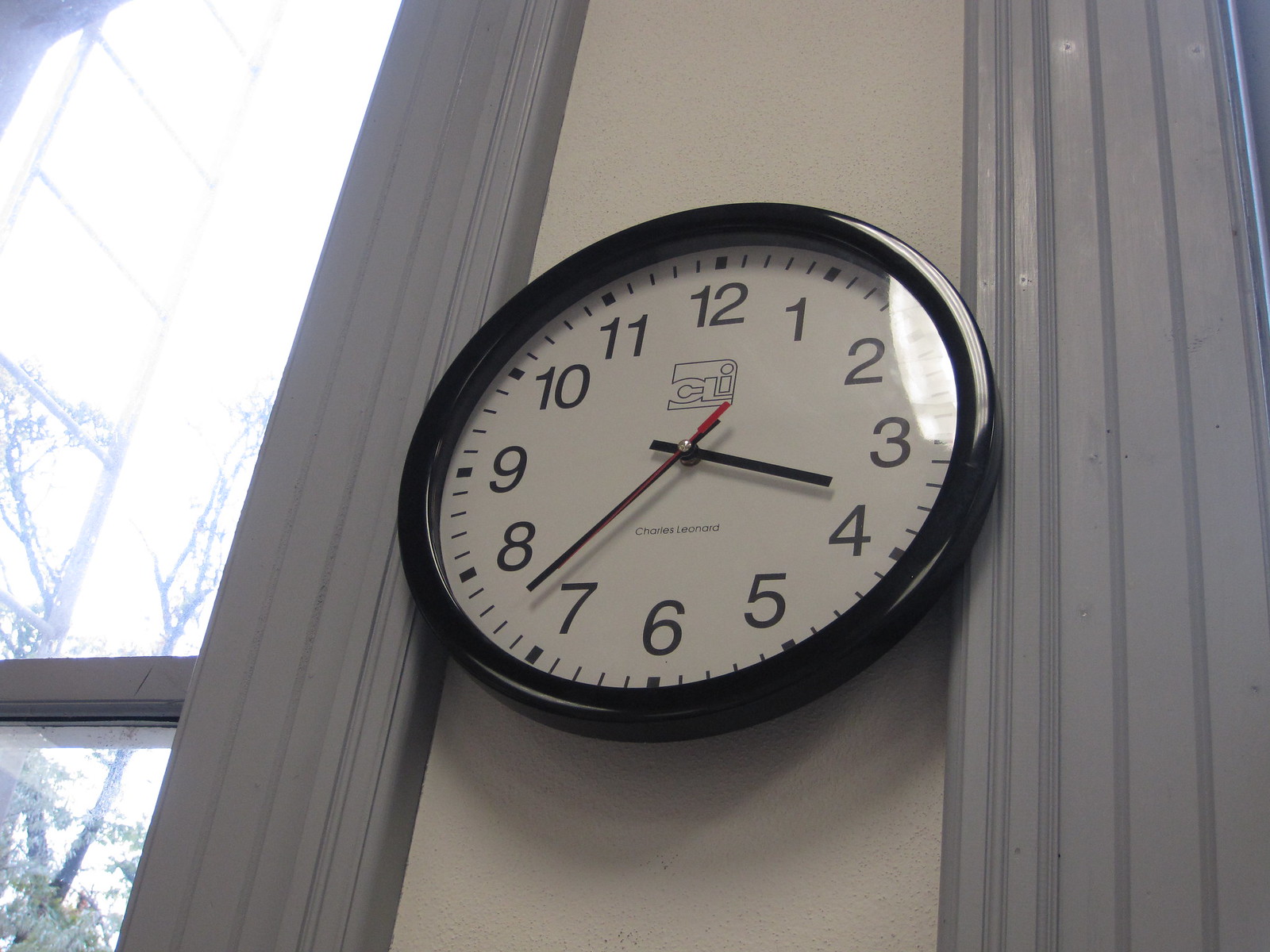This image depicts a light gray wall adorned with darker gray wooden facings, likely framing a window. Outside the window, a ladder and some foliage can be seen, illuminated by ample natural light. Between the two gray wooden frames hangs a prominent black clock made of shiny plastic, covered with a glossy glass. The clock features a white face with black numerals, two black hands, and a red second hand, indicating the time as 3:41. The overall setting is simple yet detailed, focusing on the interplay of gray tones and the striking presence of the clock.